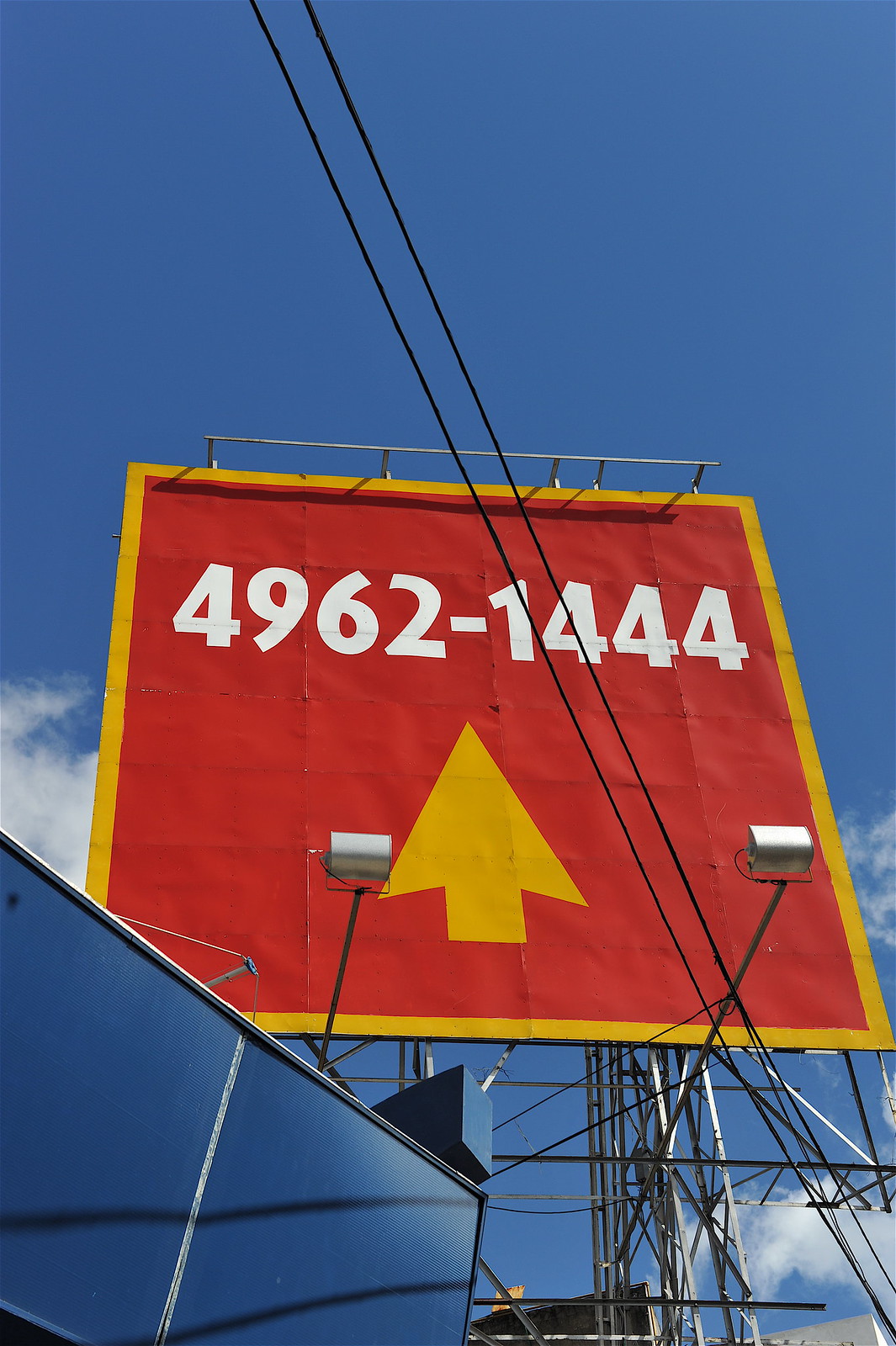The photograph captures a large, square-shaped sign situated outdoors, partially obscured by a network of electrical wires. The sign features a bold goldenrod-colored border, which frames a vibrant red interior. Centrally positioned within the red square is a matching goldenrod arrow pointing upwards. Across the top of the sign, a number sequence, "4962-1444," is prominently displayed. Behind the sign, upright metallic poles can be seen, adding to the structural elements of the scene. Reflective surfaces, possibly the side of a trailer, are visible in the background, further enhancing the composition. The sky above is a clear blue with scattered clouds, providing a picturesque backdrop to the striking sign arrangement.